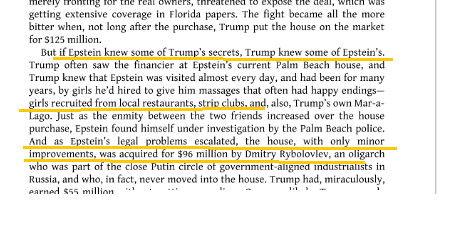The image captures a small section of text, likely from an article or digital document, focused on the tumultuous relationship between Jeffrey Epstein and Donald Trump. Key portions of the text are highlighted using a markup tool, emphasizing critical points with underlines in yellow or orange. The highlighted passages reveal details about their interactions and controversies. It notes the shared secrets between Epstein and Trump, stating, "But if Epstein knew some of Trump's secrets, Trump knew some of Epstein's." It also highlights the recruitment of girls from "local restaurants, strip clubs, and also Trump's own Mar-a-Lago," suggesting they were hired to give massages to Epstein. Furthermore, it underscores the sale of a house, acquired with only minor improvements for $96 million by Dmitri Rybolovlev, as Epstein's legal troubles escalated. This detailed snapshot offers a glimpse into the intertwined lives and scandals of the two men.